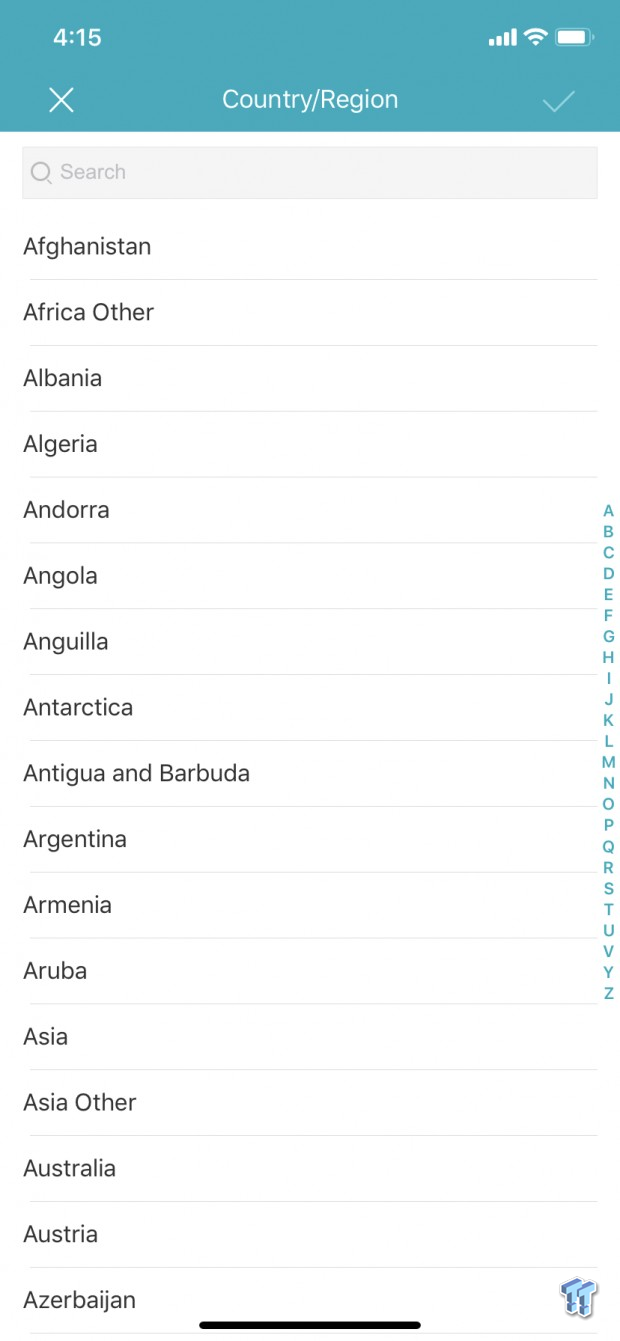A mobile phone screenshot displaying a country/region selection interface. The status bar at the top shows the current time, battery level, Wi-Fi status, and mobile connection, all presented in white font against a light blue to teal backdrop. Below this, the interface is laid out with a white background and black text. At the very top, there is a light gray search bar, just above the visible list of countries. The list is alphabetically ordered, starting with Afghanistan and ending with Azerbaijan. Users can scroll through to find their desired country. An 'X' or check mark option appears at the top of the screen to confirm the selection.